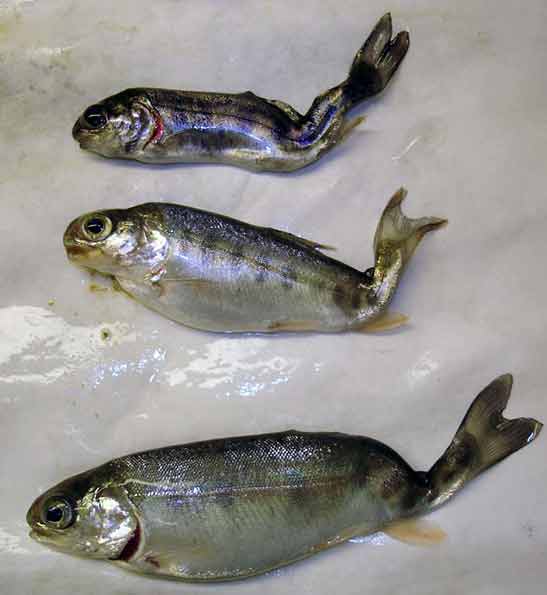This is an overhead, close-up indoor color photograph depicting three dead fish arranged side by side on a whitish surface, possibly ice, marble, or a slick, light gray stone. Their silver bodies are accented by a darker shading along their backs, with the topmost fish having a particularly pewter hue. All three fish display characteristics of rigamortis, evidenced by their slightly bent upward tails and the closed mouths. Distinguishable features include thin side fins and a small fin at the base near their tails, with no prominent upper or lower fins visible. Their eyes are black, with the middle fish having a notably larger eye. This scene is centered and devoid of any text, emphasizing its traditional photographic style.